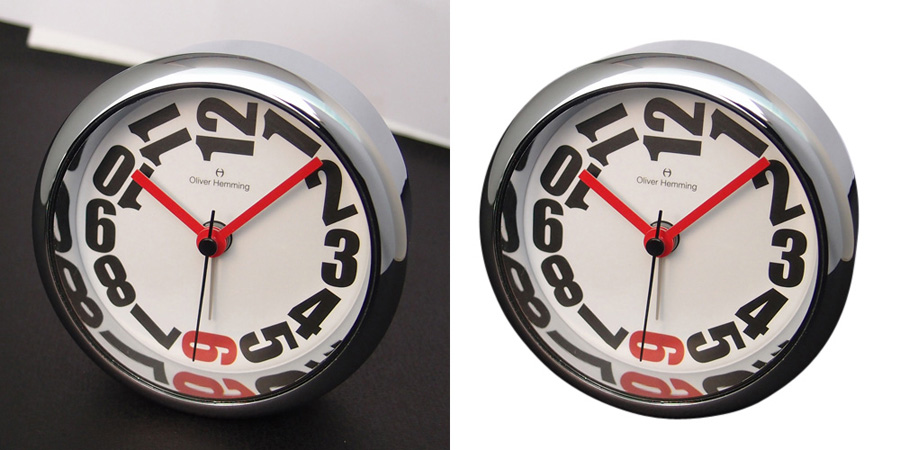The image features two identical circular clocks, each with a silver and black casing. The top half of the casing is silver while the bottom half is black. The clock faces are white with bold, black numbers from 1 through 12, but each number is uniquely tilted rather than upright, with the number 6 in red. Both clocks indicate a time of approximately 10:07. The clock hands for the hours and minutes are red, while the second hand is black. The left clock is set against a background scene with a black table surface and a black-and-white wall, giving it a real-world context. In contrast, the right clock is shown on a plain white background, similar to a marketing or online store setting, with no additional elements. Each clock features a reflection of the numbers on the bottom part of the silver frame, and they are described as being about three to four inches in diameter.